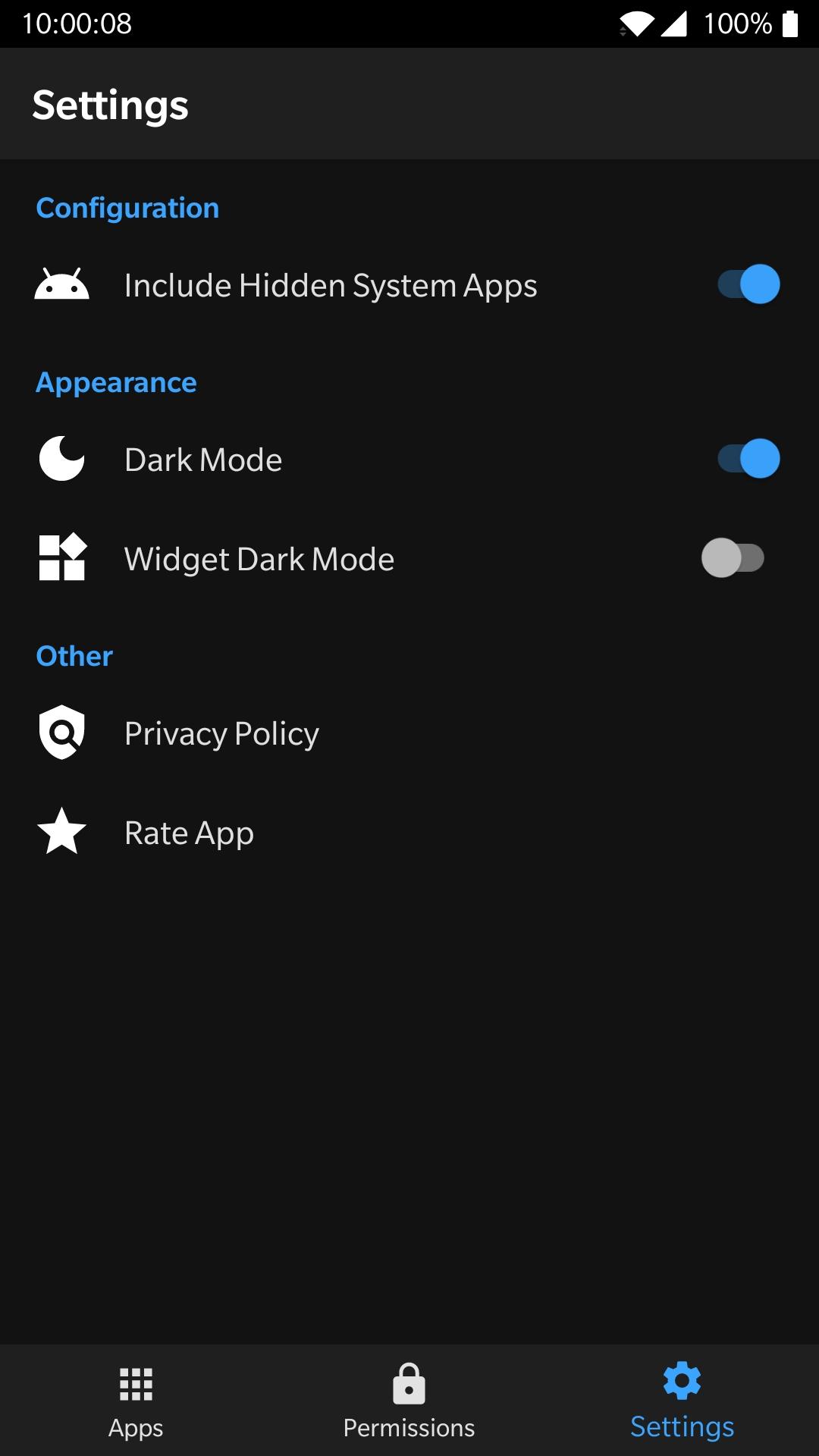The image appears to be a screenshot of a settings menu from a smartphone. The background is predominantly black. In the upper left-hand corner, a white timestamp reads "10:00:08," indicating it is either 10 o'clock and eight seconds, though it is unclear if it's a.m. or p.m. To the right of the timestamp, white icons indicate a strong Wi-Fi connection and excellent reception, with a full battery at 100%.

The screen features a dark gray border at the top, with the word "Settings" displayed in white against a black background. Below this, a blue heading reads "Configuration," followed by a white text option: "Hidden - include hidden system apps," accompanied by an oval switch with a blue circle on the right-hand side, indicating it is activated.

Further down is another blue heading, "Appearance," under which the option "Dark Mode" is displayed in white with a small white crescent icon. This is followed by a similar oval switch with a blue circle on the right, indicating an active state. Below that, the screen shows an option "Widget Dark Mode," with a graphical representation of four small rectangle icons, one of which is tilted on the upper right-hand corner, alongside a gray oval switch with the gray circle on the left, indicating it is deactivated.

The blue heading "Other" follows, listing the options "Privacy Policy" and "Rate App," the latter accompanied by a white star icon.

At the bottom of the screen, a dark gray border contains three white icons: the first labeled "Apps" with a grid of squares, the second labeled "Permissions" with a lock icon, and the third labeled "Settings" with a blue gear icon, also displayed in blue, suggesting it is the selected option.